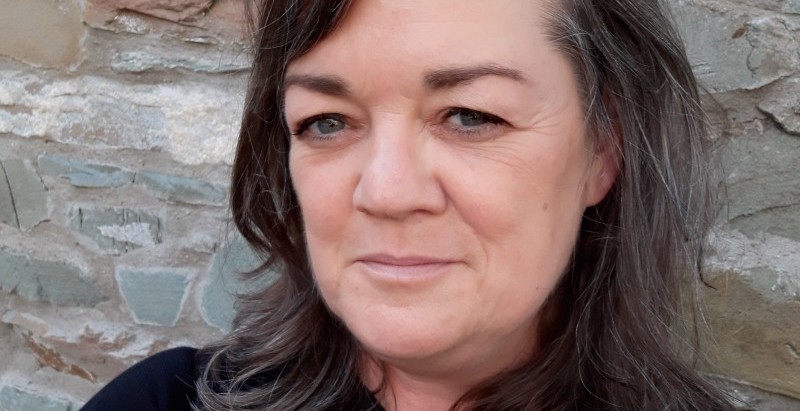This image features a middle-aged Caucasian woman, likely in her late 40s to early 60s. She has dark brown hair interspersed with gray strands, and her wide-set hazel eyes are complemented by light crow's feet and subtle wrinkles beneath them. She is leaning against a roughly textured stone wall, which comprises gray and green stones. The woman is wearing a black shirt and is giving a slight smile, possibly a smirk, while looking directly into the camera. Her expression and the stone backdrop suggest that this could be a profile photo with a somewhat professional appearance.